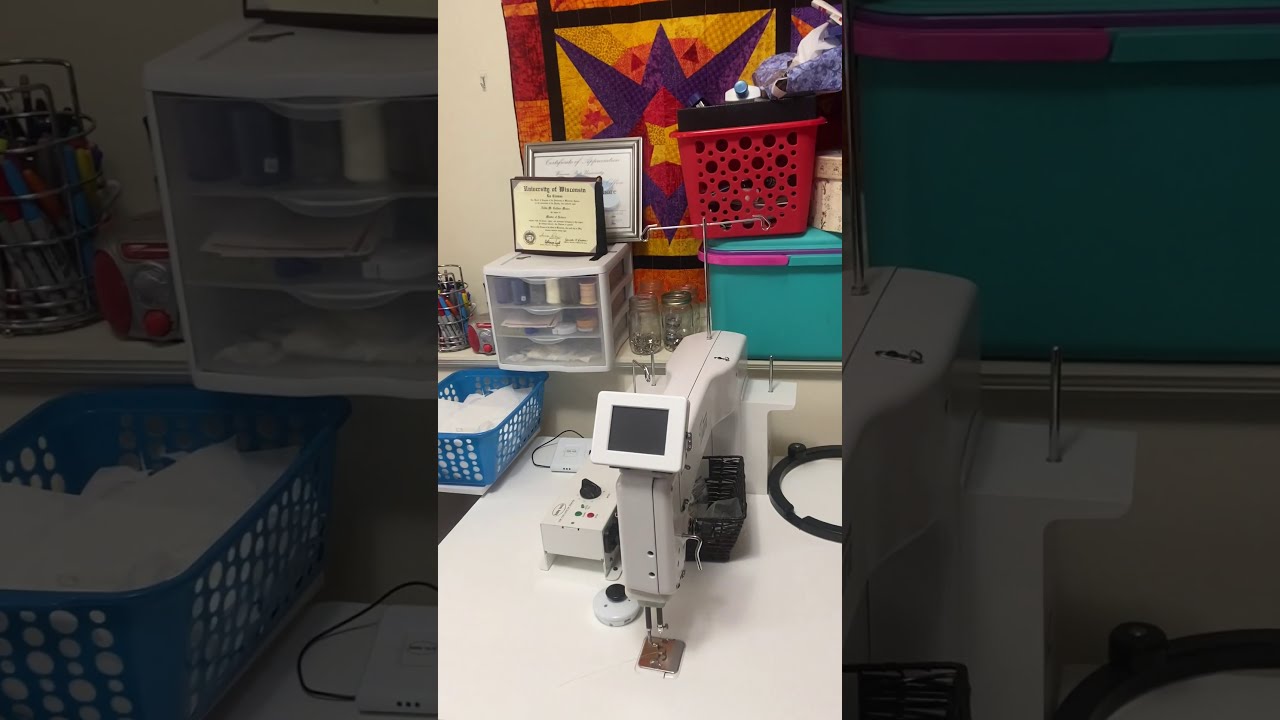This image is a detailed photograph of a white electronic sewing machine positioned centrally on a white table. The sewing machine features a small screen for displaying information, and the photograph appears to be taken with a cell phone, evident by the bright center framing surrounded by a grayed-out background. To the left of the sewing machine is a blue plastic basket, likely filled with white cotton or paper.

In the background, a white wall supports multiple shelves and containers. One shelf holds two baskets, two glass jars, and a pen holder. Below the shelf, there's a red plastic tub stacked on a teal plastic tub. Adjacent to these is a turquoise container with a closed top. 

The wall also features several framed certificates and awards. Among these, a diploma from the University of Wisconsin stands out, along with a certificate of appreciation in a silver frame.

Centrally mounted on the wall is a vibrant quilt decorated in shades of red, orange, yellow, and purple. The quilt's design includes a black square at its center, surrounded by a purple star with projecting points, and layers of red and yellow radiating outward. This intricate quilt adds a pop of color and artistry to the scene.

Overall, the photograph captures an eclectic and organized workspace, rich in colors and busy with various tools and recognitions, hinting at someone's sewing and crafting hobby or profession.